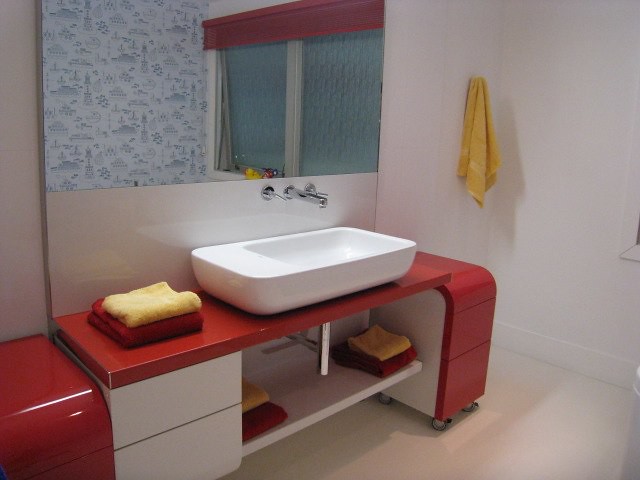This bathroom portrait features a vibrant and organized space characterized by a distinctive red-and-white color palette. On the left side of the image, there is a sleek, red glossy countertop that supports a standalone white sink with a silver faucet extending from the wall above. Underneath the sink sit two white cabinets, stacked on top of each other, providing functional storage space. 

Adjacent to the cabinets, in the left corner of the room, stands a red glossy item, possibly a toilet or a trash receptacle, adding a pop of color to the scene. The right side of the photograph showcases a red, glossy two-drawer standalone cabinet with a distinctive downwardly curved top, supported by four wheels for easy mobility. 

The center of attention, the white sink, rests on the red countertop and is adorned with rags—yellow on top of red—placed neatly to the left and right underneath it, with a similar arrangement on the countertop next to the sink. Above the sink, a large rectangular mirror reflects part of the bathroom, revealing a cityscape-patterned shower curtain and two frosted rectangular windows with a red blind set at the top. 

Completing the vibrant decor, a yellow towel is tastefully hung on the wall in the corner of the room. The white walls and floor provide a crisp, clean backdrop that enhances the striking red-and-yellow accents throughout the bathroom.